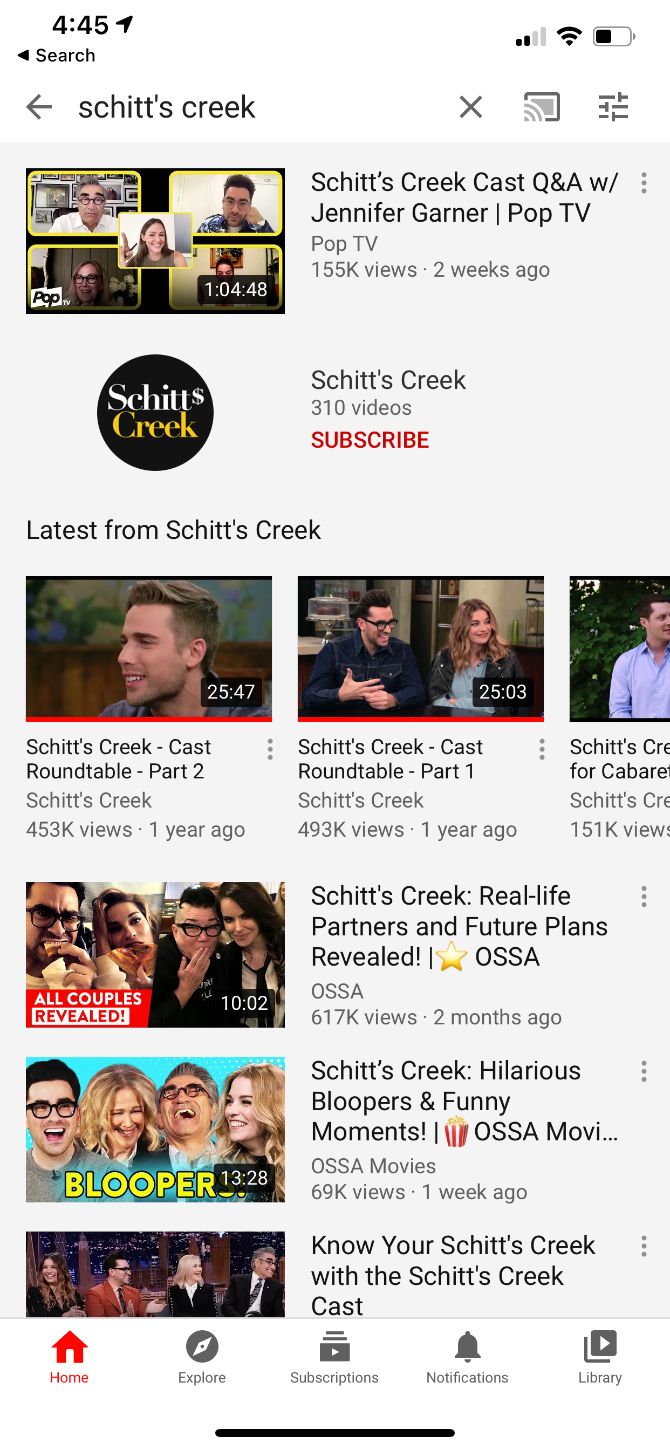A screenshot of a cell phone display features a detailed overview of a Schitt's Creek-focused page. At the top, the heading prominently reads "Schitt's Creek," stylized as S-C-H-I-T-T-'s Creek. The central feature is a highlighted video titled "Schitt's Creek's Cast Question and Answer with Jennifer Garner, Pop-Up TV," lasting an hour, four minutes, and 48 seconds. Below this, there is an option to subscribe, showing the channel has 310 videos, with a bold red "subscribe" button beneath it.

The section labeled "Latest from Schitt's Creek" includes three thumbnail videos aligned horizontally, followed by another row of three more videos in a similar arrangement. The top two videos each have a runtime of approximately 25 minutes. Further down, the content includes entertaining bloopers, insights into future plans for the cast, and a segment titled "Know Your Schitt's Creek with the Schitt's Creek Cast." Each video listing has accompanying information displayed to the right of the thumbnails, making it easy to distinguish between the different types of content available.